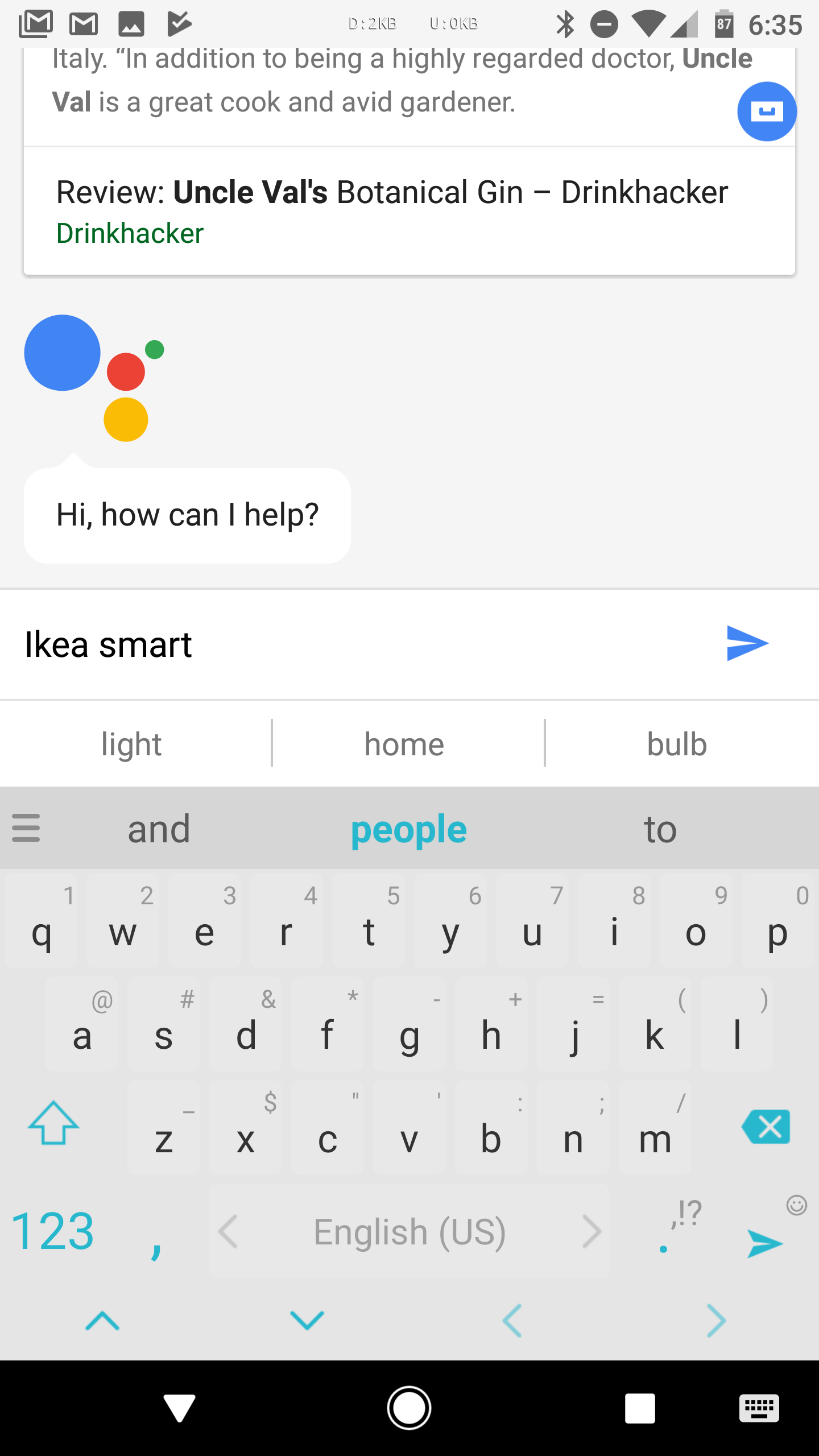This image is a screenshot captured from a smartphone, detailing a user's interaction with a digital assistant app, potentially Google Assistant. The top of the screen shows various status icons including an 'M' icon, Bluetooth symbol, Wi-Fi signal, the current time (6:35), and the battery level (87%). 

The main portion of the display shows a white interface with partially visible text at the top that reads, "Italy In addition to being a highly regarded doctor, Uncle Val is a great cook and avid gardener." Below this text, there is a blue link button that appears to say, "Review Uncle Val's Botanical Gin - Drink Hacker," with the 'Bot' partially cut off. Next to this link, four small colored circles (blue, red, green, and yellow) are positioned, likely representing the Google Assistant's colors.

Prominently displayed below is a greeting from the assistant saying, "Hi, how can I help?" Just beneath this, the user is in the process of typing "IKEA smart" into the chat box. The message is accompanied by a send button on the right of the text input field.

The screen also shows the smartphone's virtual keyboard, featuring predictive text suggestions including "light," "home," and "bulb." The partly visible keyboard keys include words like "and," "people," and "two." At the bottom of the screen are typical navigation buttons: a keyboard switch button, a home button, and other standard controls.

Overall, it captures a moment of the user engaging with their digital assistant, requesting information related to "IKEA smart" products.